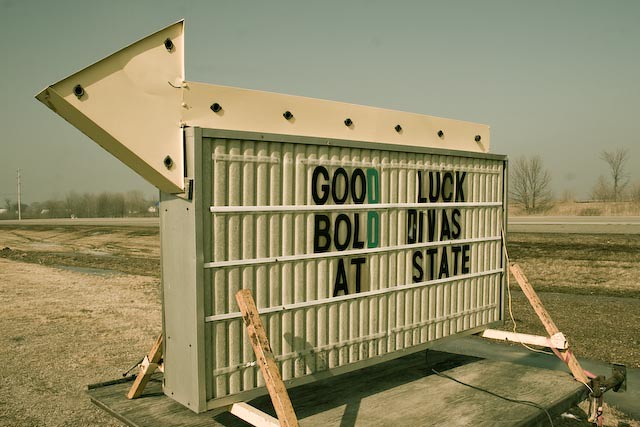The image depicts an old-style reader board or marquee sign lying on the ground, supported by fresh wooden pegs and resting on a concrete slab. The sign, which appears to be in a desolate, sparsely wooded area with dried-out grass and leafless trees, reads "Good Luck Bold Divas at State" in black letters, with the 'D' in 'Good' and 'Bold' highlighted in green. A large arrow pointing to the left sits atop the sign, featuring circular spots likely meant for lights to illuminate the direction. Beyond the sign, a small two-lane road is visible in the background, accompanied by a telephone pole on the lower-left side. The cloudy sky adds to the overall barren and remote atmosphere of the scene.